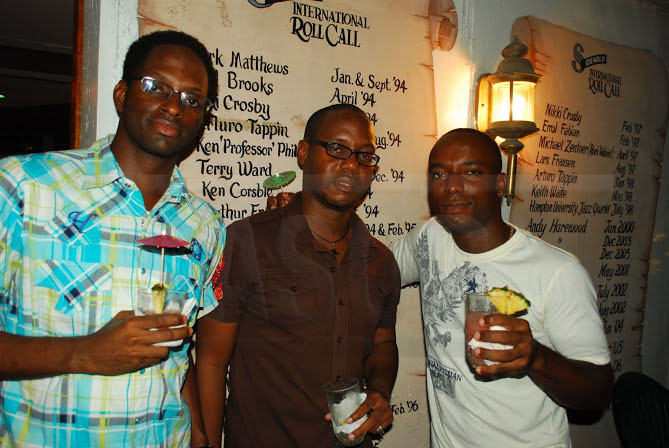In a lively bar, three black men in their late 20s or 30s stand together, each holding a cocktail. On the left, the tallest man wears a short-sleeved, plaid button-down shirt in shades of blue, green, and white. He sports glasses, is clean-shaven with short black hair, and holds a drink adorned with a small umbrella and a pineapple slice. The man in the middle, also clean-shaven with black-rimmed glasses and short hair, wears a brown button-up short-sleeve shirt and clutches his drink in his left hand. The man on the right is in a white graphic t-shirt, smiling at the camera with his left hand holding a drink garnished with a pineapple wedge and his right hand resting on the middle man's shoulder. Behind them, a white wall features two large signboards designed like old parchment scrolls, titled "International Roll Call," listing names and dates from various years. The scrolls include partial names and dates like "Matthews, Jan September 94" and "Nicky, Crosby Feb 97." A lit lamp hangs between these scrolls, adding a warm glow to the scene. The background beyond an open door is dark, contrasting with the well-lit camaraderie of the three friends in the forefront.